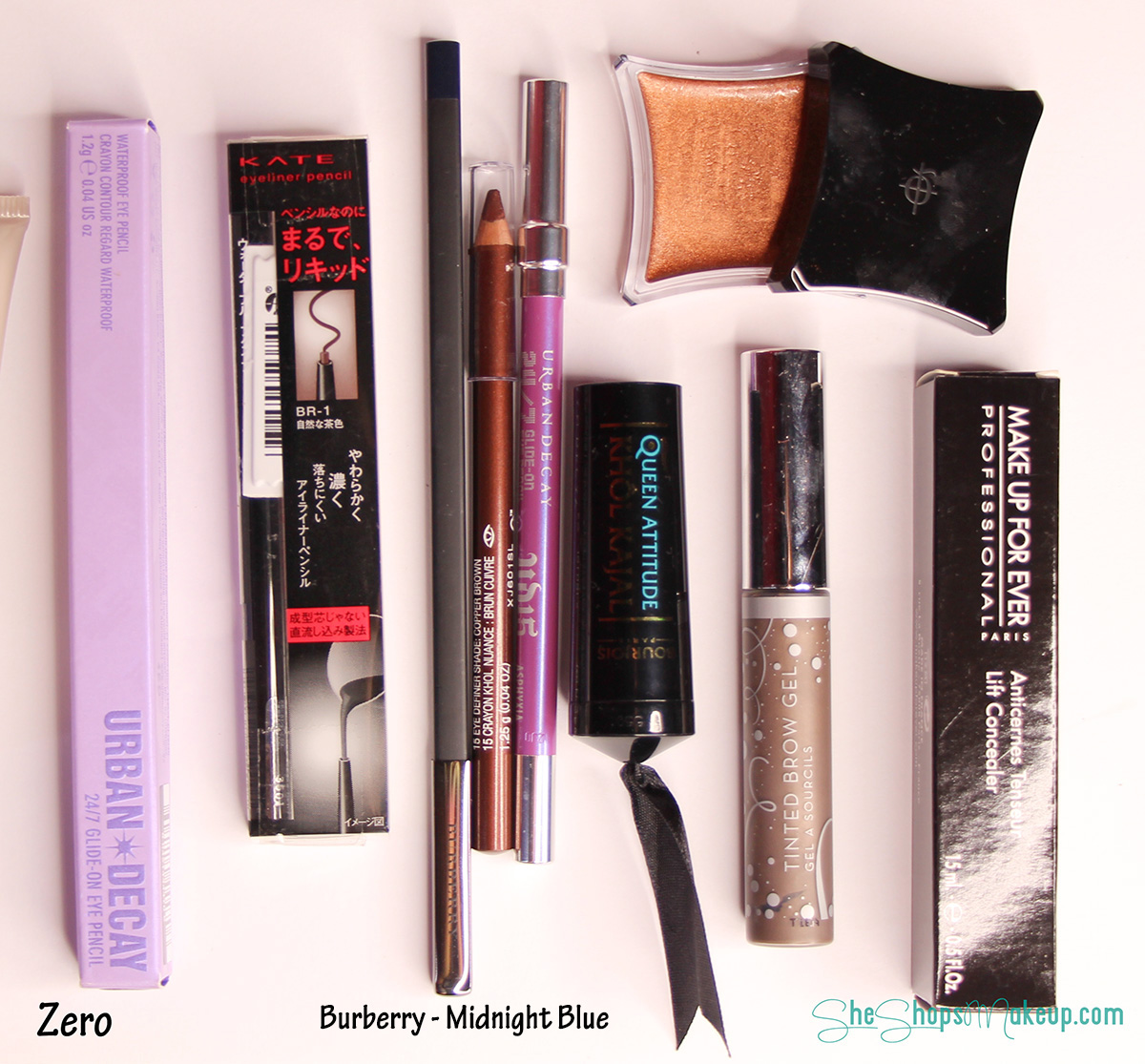This photograph features an array of makeup products meticulously arranged on a table. The selection includes a variety of items essential for a complete makeup routine. On the far left, there is an eyeliner from Urban Decay. Next to it is a makeup stick branded with the name "Kate," adorned with distinctive red Asian lettering on the packaging. Moving right, there is an eyeliner or potentially a lip liner in the shade Burberry Midnight Blue. Adjacent to that is a compact of powder or foundation. Additionally, there is a Forever Anti-Tensor Lift Concealer and a tinted brow gel. The collection is rounded off with another eyeliner or possibly mascara. The presence of the websites SheShopsMakeup.com and Makeup Professionals is noted among the items, suggesting sources or brand affiliations. This image, devoid of any distracting background elements, focuses solely on the makeup products.